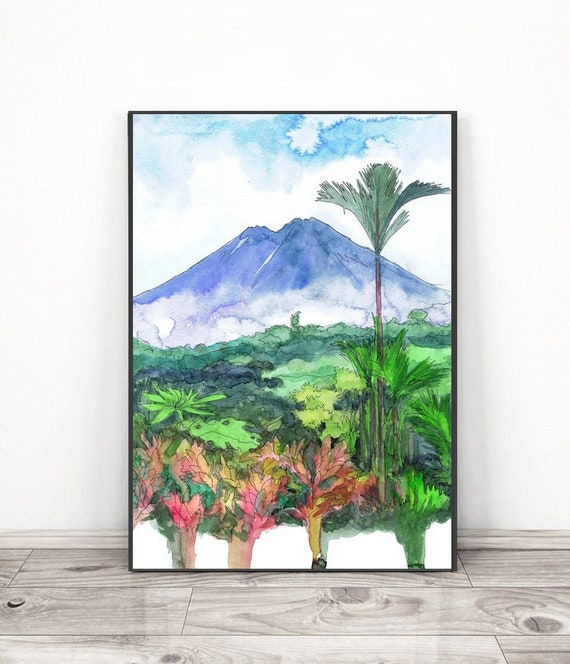This is a detailed photograph of a large watercolor painting encased in a black frame, leaning against a pristine white wall with a faux wood gray and white patterned floor beneath it. The painting vividly depicts a tropical scene, possibly reminiscent of Hawaii or Polynesia, featuring a towering, blueish mountain that could be an inactive volcano. The sky above is an aqua blue watercolor wash, with wisps of white clouds creating a misty effect around the volcano’s base, giving the illusion that it is above the clouds. Dominating the foreground is a tall, solitary palm tree, its leafy crown extending high above the rest of the vegetation. The surrounding foliage is a vibrant mix of various shades of green, from lime to deep forest green, interspersed with tropical flowering plants in shades of pink, yellow, and red. The lush greenery and colorful flowers, including purples and vivid limey greens, create a rich tapestry of tropical life, making the scene both lively and tranquil. The painting is unsigned and text-free, inviting viewers to immerse themselves in the serene tropical landscape it portrays.